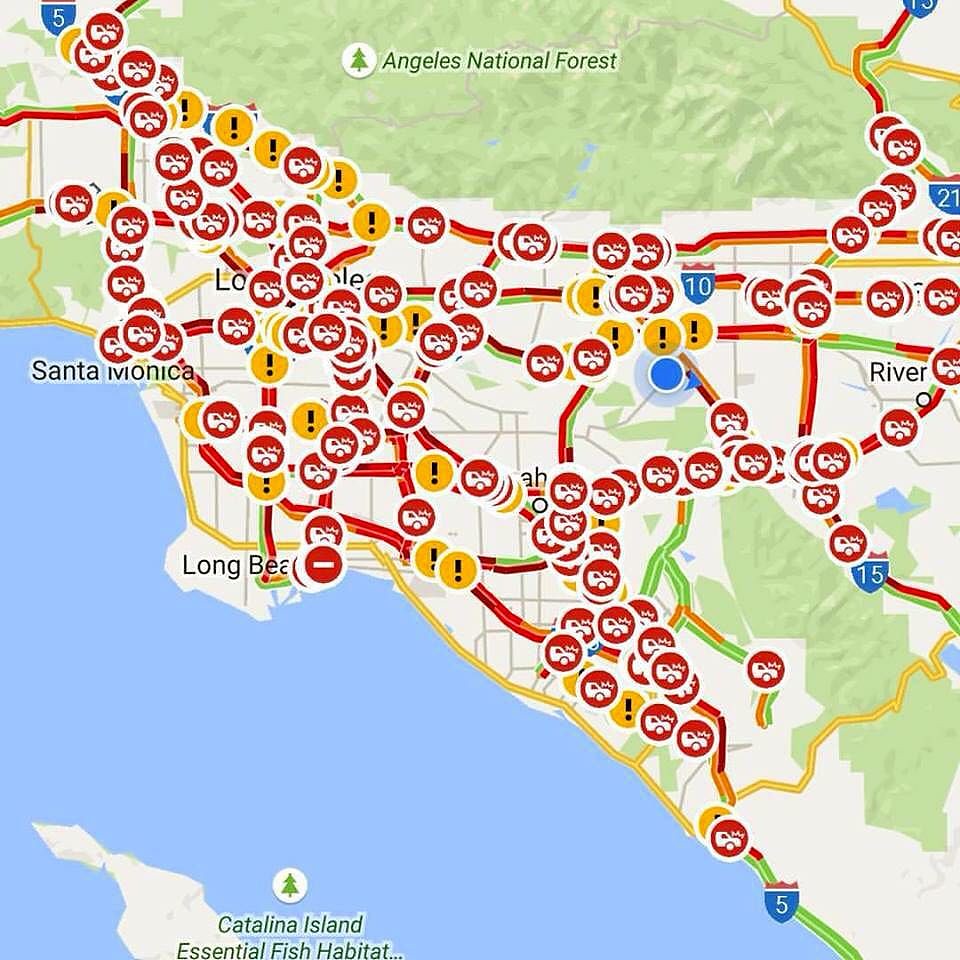This is a detailed screen capture of a traffic map focusing on the Los Angeles metropolitan area, including prominent locations such as Long Beach, Santa Monica, and Riverside. The map highlights several major routes—such as Route 5, Route 10, Route 15, and Route 21—all represented with their respective color-coding: blue for routes with red tops and white numbers. At the top of the map, the Angeles National Forest is depicted in a green area with its name in green font next to an evergreen tree symbol. 

In the bottom left corner, the coast of California is visible, extending up the left side, delineating the boundary with the Pacific Ocean. Catalina Island is marked near the bottom with a green label indicating it as an essential fish habitat, accompanied by a tree icon within a white circle.

The map is dense with traffic indicators: red and yellow lines on the highways denote varying levels of traffic congestion, with red indicating severe delays. Numerous red symbols representing vehicle collisions, identified by silhouettes of cars with emanating triangle signs, are scattered across the map. Yellow circles with black exclamation points indicate cautions or warnings in specific areas. Some locations are labeled in black font, such as Los Angeles at the top, and other regional towns.

The map presents a clear depiction of the significant traffic and accident spots within this area of California, capturing a snapshot of the transportation conditions and illustrated caution areas effectively.